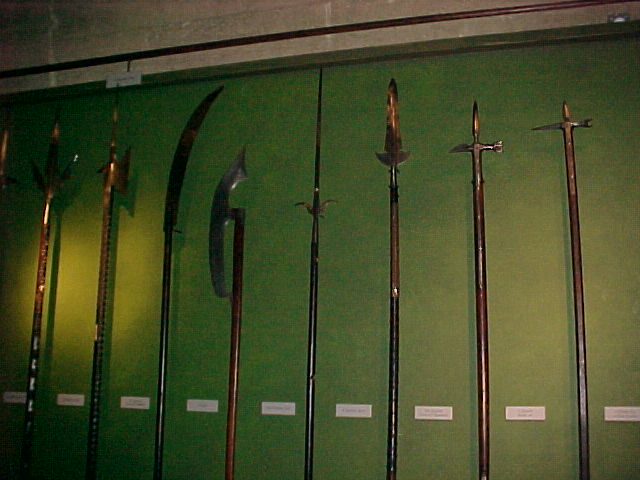The color photograph in landscape orientation showcases a museum display with medieval weapons elegantly mounted against an olive green background, set into a brown and white, possibly marble wall. The display features eight distinct weapons, each meticulously placed in its own section. Among the implements are swords, spears, and what appear to be multi-pronged spears and a scythe. Prominently, a very narrow and sharp spear extends to the top of the approximately six-foot-tall display, with the weapons varying in length from around four to five and a half feet. One weapon appears bent at the end, contrasting the generally straight and sharp-ended others, some of which sport cross-guards. Under each weapon is a small white placard with descriptions, though the text is not legible in the photograph. The display, characterized by photographic realism, suggests a historical exhibition, possibly in a museum, offering insights into the design and use of these medieval armaments.